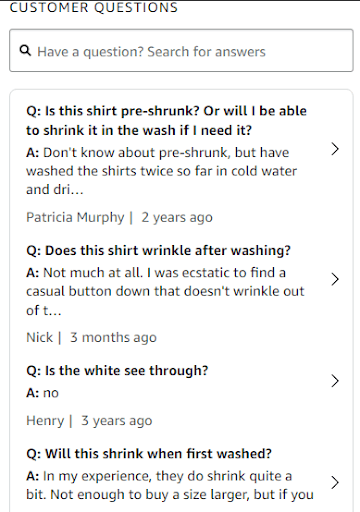The image appears to be a screenshot resembling an Amazon webpage, specifically the Customer Questions & Answers section often found on product listings. However, there is no explicit Amazon branding visible to confirm this. The webpage displays a series of questions and answers attributed to various customers:

1. **Question**: "Is the shirt pre-shrunk or will I be able to shrink it in the wash if needed?"  
   **Answer**: "Don't know about pre-shrunk, but I have washed the shirt twice so far in cold water, and then..." — **Patricia Murphy**, two years ago.

2. **Question**: "Does this shirt wrinkle after washing?"  
   **Answer**: "Not much at all. I was ecstatic to find a casual button-down that doesn't wrinkle out, and then..." — **Nick**, three months ago.

3. **Question**: "Is the white tee see-through?"  
   **Answer**: "No." — **Henry**, three years ago.

4. **Question**: "Will this shrink when first washed?"  
   **Answer**: "In my experience, they do not shrink quite a bit. Not sure to buy a size larger, but if you..." *(answer truncated)*.

At the top of the screen, there is a search bar labeled "Have a question? Search for answers," allowing users to type in their queries to see if they have already been addressed by previous customers.